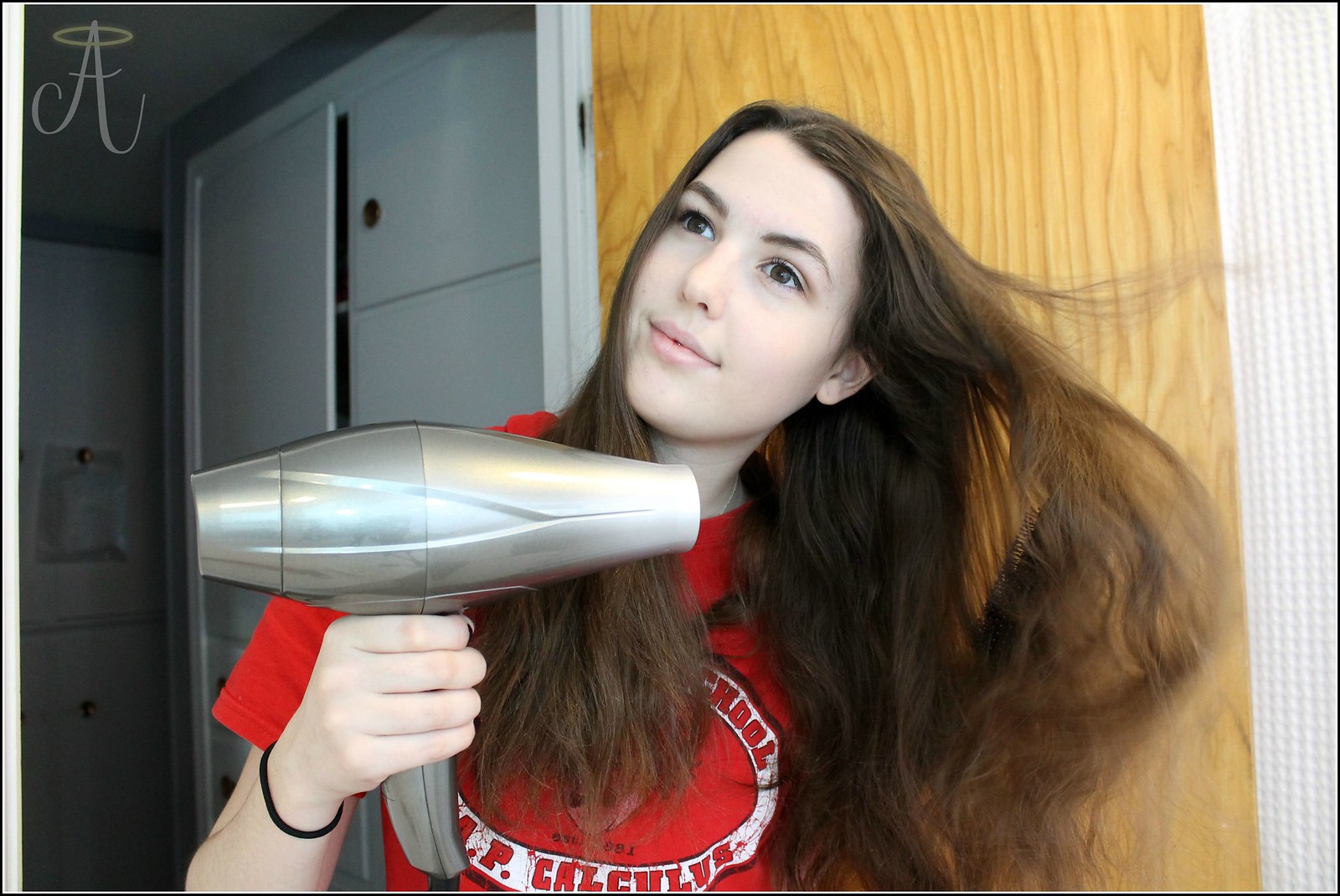This indoor color photograph, oriented horizontally, features a close-up portrait of a young girl, approximately 16 to 20 years old, standing at the center. She has long brunette hair that streams behind her, blown by the silver hairdryer she holds in her right hand. Her head is slightly tilted up and to the right, with a subtly upward gaze. Clad in a red t-shirt adorned with some type of logo, she also wears a black rubber band around her right wrist. The backdrop consists of a light wooden panel, with a dimly lit room containing tall white cabinets visible to the left. Notably, a capital letter "A" with a halo is superimposed in the top left corner of the image. A thin black line border frames the entire photograph.